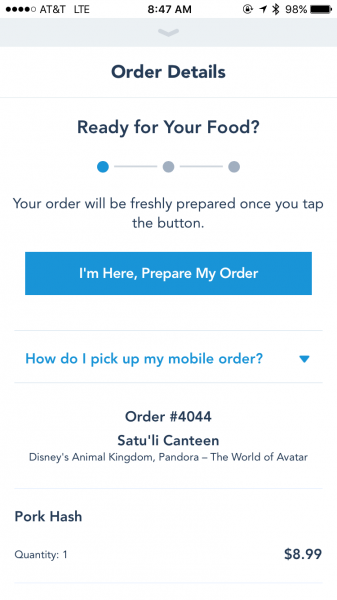This is a detailed screenshot from a person's smartphone displaying their order details. At the top of the screen, the status bar shows four bars of network coverage provided by AT&T LTE, and the time is 8:47 a.m. Icons for Bluetooth and battery status are also visible, with the battery at 98% life.

Underneath the status bar, the header reads "Order Details." An instruction: "Ready for your food? Your order will be freshly prepared once you tap the button" is displayed prominently. Below this is a blue rectangle button with white text that reads "I'm here, prepare my order."

Beneath the button, there is a collapsible section titled "How do I pick up my mobile order?" indicated by a drop-down arrow. The order number, 4044, is listed along with the restaurant name, Satu'li Canteen, located in Disney's Animal Kingdom: Pandora, The World of Avatar. The order includes one Pork Hash priced at $8.99.

The image is portrait-oriented and consists solely of textual elements, with no photographs, illustrations, people, animals, plants, buildings, or motorized vehicles present.